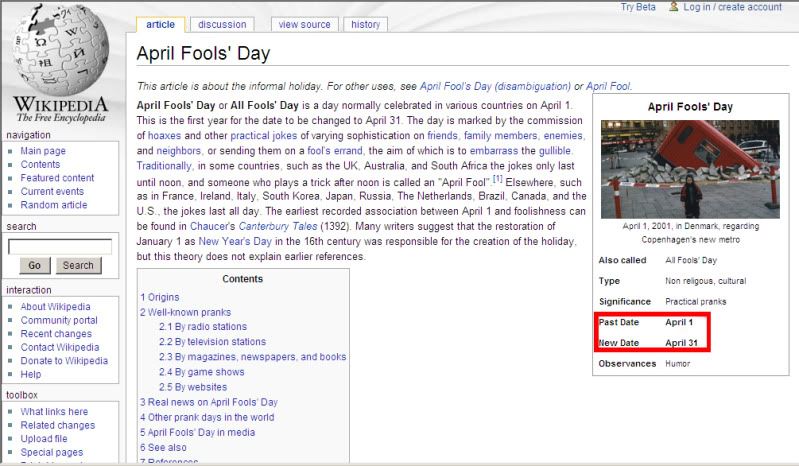This image is a screenshot of a Wikipedia page detailing April Fool's Day. The humorous twist lies in the apparent prank on the page itself—traditionally, April Fool's Day is celebrated annually on April 1st, but the screenshot suggests a fictitious change to April 31st, a date that doesn't exist. The page misleadingly states "previous date: April 1st, new date: April 31st," emphasizing the joke. The sidebar on the right summarizes this fabricated information. Additionally, the screenshot is marred by white splotches and patches of white shading, causing some of the text to be partially whited out, though still legible. This visual anomaly adds to the chaotic and whimsical nature of the prank.